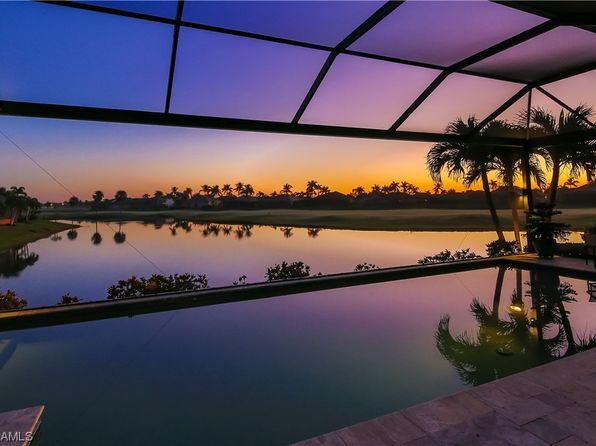In this image, you're presented with a tranquil view of a long rectangular swimming pool situated in a tropical setting during sunset. The pool is surrounded by gray stone pavers and has a clear, see-through canopy with a distinctive V-shaped arch, allowing an unobstructed view of the vivid sky above. The sky is a breathtaking display of purples, blues, and oranges as the sun sets. Palm trees are positioned close to the pool, casting dark silhouettes and their reflections dance on the water’s surface, which shimmers in hues of purple, blue, and green. Beyond the pool, there's a serene natural body of water, possibly a river or lake, mirroring the colorful sky and distant palm trees. The setting is serene and picturesque with additional trees and bushes separating the pool area from the water, completing the tropical atmosphere.